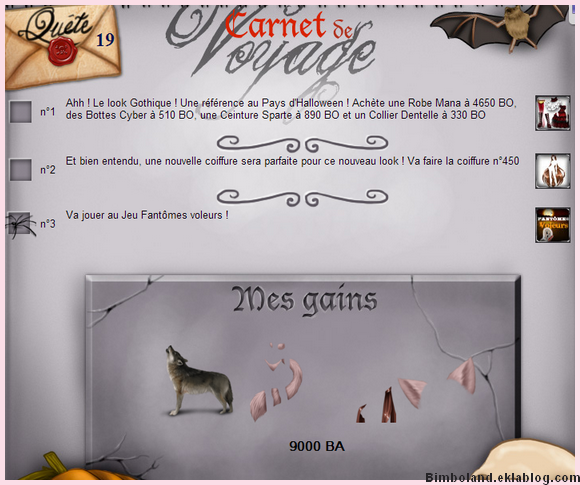The screenshot, likely from a video game, features a predominantly gray background with intricate details that hint at a narrative or quest. At the very top, the title "Carnet de Voyage" is displayed, with "Carnet" in red and "Voyage" in dark gray. In the upper left-hand corner, there is an antique yellow envelope adorned with a red wax seal impressing the number "19" to the side and the cursive word "Quête" above it. On the right-hand corner, a bat with its wings spread is depicted. 

The center part of the image is filled with three sequentially numbered sections, each accompanied by small French text, suggestive of a storyline or objectives. Adjacent to these sections are pictorial icons instead of traditional check marks—one notably featuring a spider. 

Towards the bottom of the image, captions in dark gray mention "Mess Gains" and "9000 B.A.," possibly indicating an achievement or an upgrade. Illustrations nearby depict a wolf and fragmented bone graphics, suggesting a thematic connection to the character's journey. The overall aesthetic includes subtle line textures to give a cracked appearance, enriching the visual complexity of the screenshot.